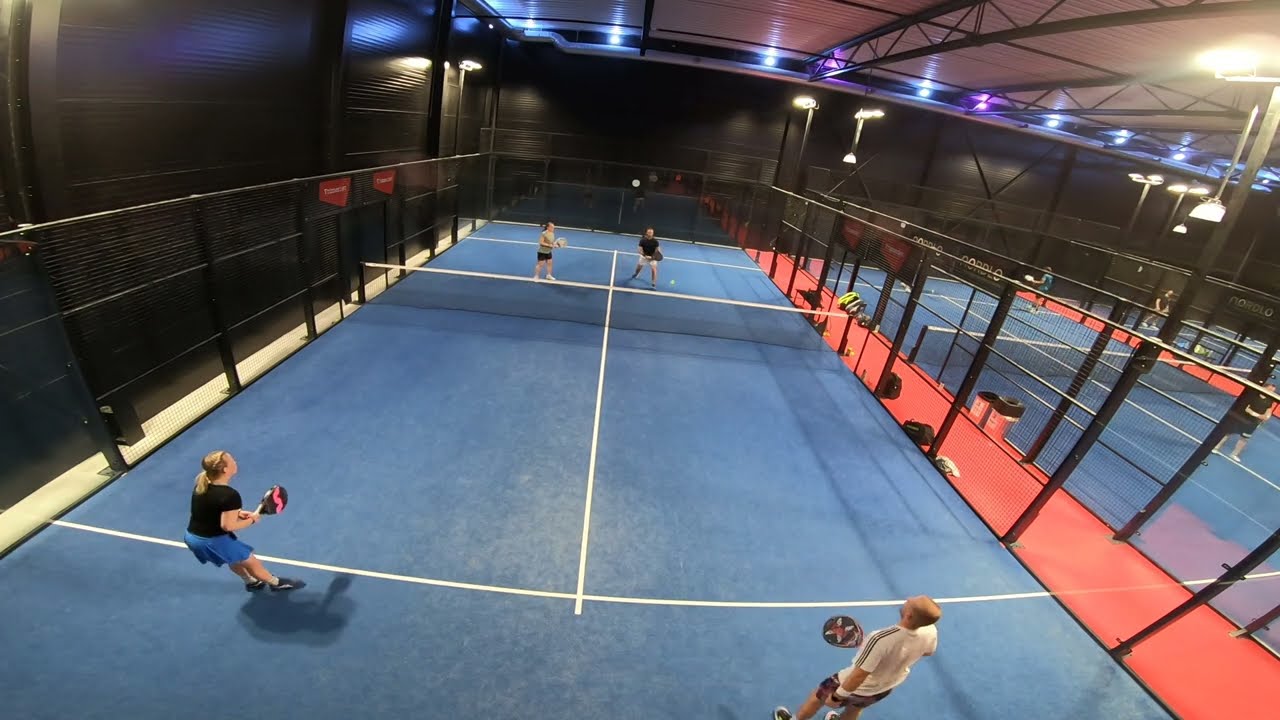This detailed wide rectangular photograph captures an indoor tennis court setting from a high vantage point, possibly a balcony. The foreground features the short edge of a vibrant blue tennis court marked with white paint, extending towards the horizon line at the back of the image. Two individuals are prominently standing behind the white baseline: on the left, a blonde white woman dressed in a blue skirt and black shirt, and to the right, a blonde white man clad in a white shirt and shorts. Positioned behind the central net, centrally to the court, a young girl in a gray shirt and shorts prepares to play, while a man in a black shirt and white shorts stands to her right.

Surrounding the court is a red walkway, which transitions into additional tennis courts observable to the right-hand side of the image. The courts are separated by black fencing and nets. The entire arena is brightly lit with a mix of blue and purple lights, contributing to a well-illuminated environment. The ceiling is white, and at the back of the court, a black wall can be seen. The photograph offers a comprehensive view of a lively indoor tennis match with multiple players presumably engaged in a doubles game, all holding rackets and poised in their respective stances.